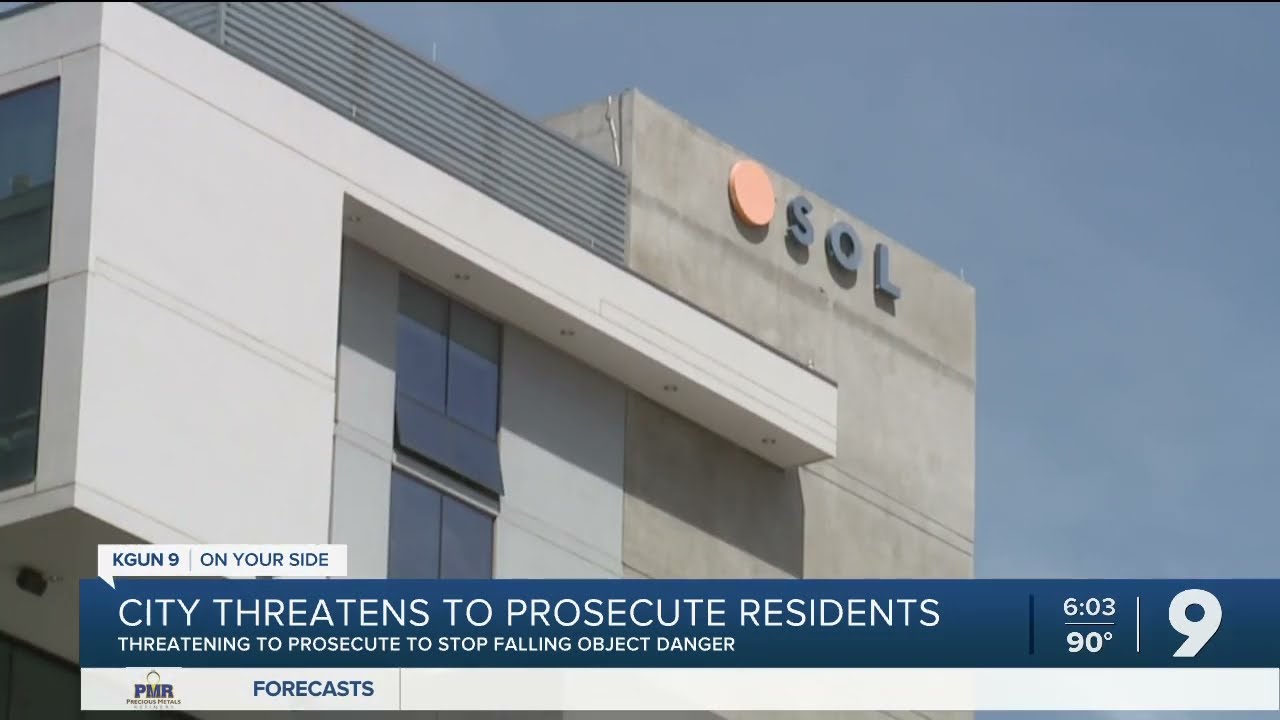This image is a detailed screenshot from a local news broadcast on KGUN9, On Your Side. The photograph captures the side of a large, gray concrete building with white walls and black windows. Prominently displayed on the upper right side of the building is an orange circle accompanied by the letters "SOL" in dark gray, indicating the name or logo of the company. The background features a clear blue sky, suggesting the image was taken during the daytime with no clouds visible.

At the bottom of the image, there's a prominent blue news banner over a white stripe. The blue banner includes the KGUN9 logo, the current time of 6:03, and a temperature of 90 degrees. It also contains the headline: "City threatens to prosecute residents. Threatening to prosecute to stop falling object danger." Adjacent to this on the white stripe are the letters "PMR" in black and the word "forecasts" in blue, reinforcing the broadcast's local news context.